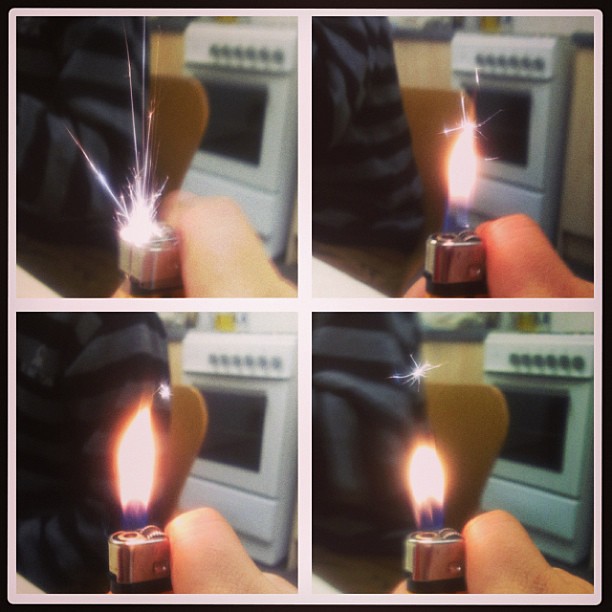This image is a composite of four photographs capturing the process of lighting a black Bic lighter. In each square, the images transition from initial spark to diminishing flame. 

In the first photograph, an individual wearing a gray sweatshirt with black stripes is seated in a light brown wooden chair. They flick the black lighter, causing bright sparks to fly up. To the right, the white stove with brown knobs and a black oven window is visible, along with wooden cabinets in the background.

The second photograph shows the lighter’s flame starting to rise. This flame is colorful: blue at the bottom, transitioning to white in the middle, and finally orange at the top, with a few sparks at the very peak.

In the third image, the flame is fully developed, displaying the same gradient of blue, white, and orange. The background remains consistent with the stove and cabinets.

The final photograph captures the flame diminishing to about half its previous size. The person’s thumb is still pressing down on the lighter, and there is a faint spark visible at the top. The overall scene, with the stove and cabinets, remains unchanged, creating a cohesive narrative of the lighter-igniting process.